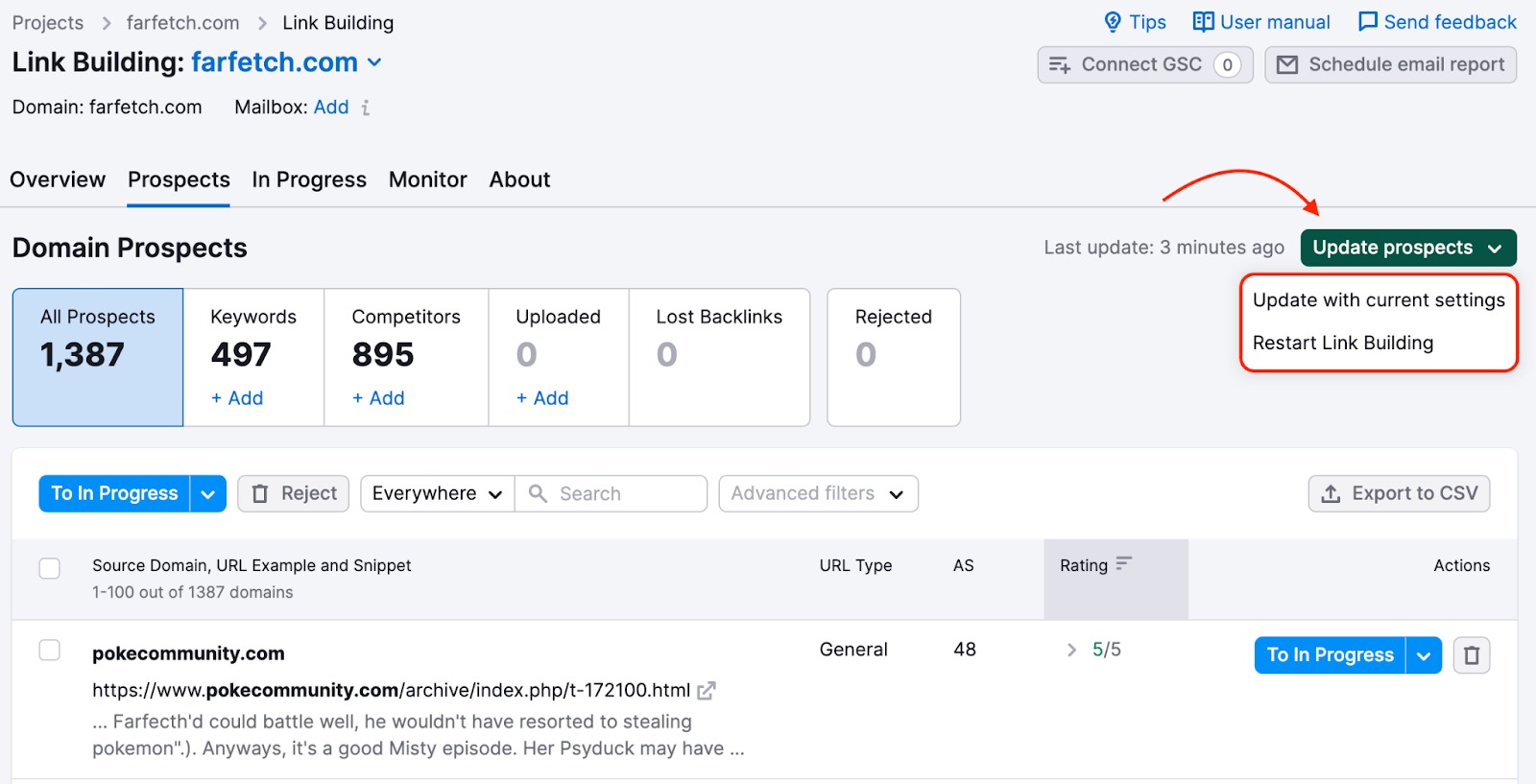This is a detailed screenshot of a web page on Farfetch.com, a domain dedicated to a project titled "Link Building." The navigation breadcrumbs at the top left reveal the user's journey from "Projects" to "Farfetch.com" and finally to the "Link Building" section. The domain displayed is consistently Farfetch.com.

In the main workspace, notable sections are divided into several tabs: "Overview," which is currently active, indicated by a dark black highlight and a dark blue underline, along with other tabs labeled "In Progress," "Monitor," and "About." Directly below these tabs is the "Mailbox" section, which currently displays an option to "Add," suggesting no mailbox has been configured yet.

The top right part of the screenshot features additional tabs for user assistance, including "Tips," "User Manual," and "Send Feedback," providing resources for users needing help with website design or other functionalities. Also in this area, a timestamp reading "Last Update three minutes ago" is connected by a red curved arrow to a button labeled "Update Prospects." Clicking this button reveals a pop-up box with options to "Update with current settings" or "Restart Link Building."

The "Domain Prospects" section below presents detailed metrics: "All Prospects" numbered at 1,087, "Keywords" at 497, "Competitors" at 895, while “Uploaded,” "Lost Backlinks," and "Rejected" all stand at zero, indicating these sections are either new or inactive.